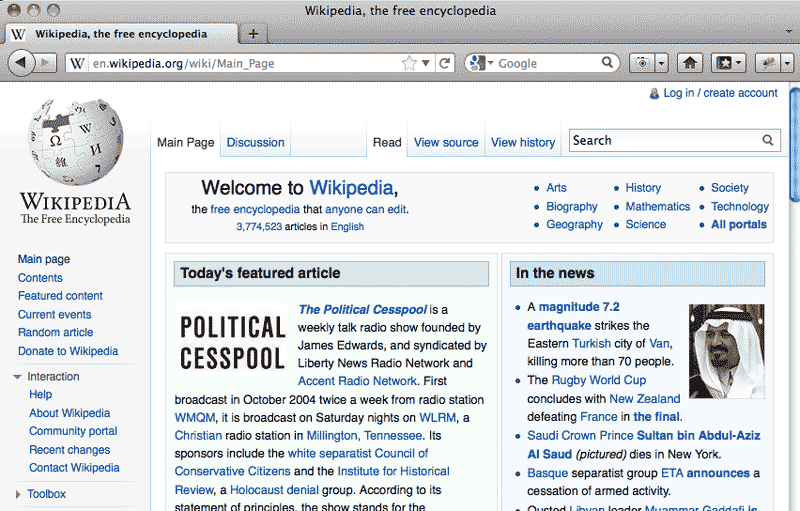This screenshot captures the main page of Wikipedia, viewed through the Google Chrome browser, which is identifiable by the characteristic three vertical dots in the top-right corner of the browser window. The URL bar at the top indicates the webpage being displayed is "wikipedia.org" with "Main Page" specified in the URL, confirming it as Wikipedia's primary landing page.

In the browser's top interface, beside the URL bar, there is a Google search bar on the right, followed by several icons including, noticeably, the home button. The left sidebar of the webpage shows the standard navigation menu found on Wikipedia, listing options such as "Main page," "Contents," "Featured content," "Current events," "Random article," and "Donate to Wikipedia."

The central portion of the page showcases "Today's featured article," which is currently discussing a topic from "The Political Cesspool." Adjacent to this section, on the right side, is an "In the news" section that presents a selection of short news summaries with brief descriptions of current events. The overall layout and design elements are consistent with Wikipedia's typical aesthetic, emphasizing easy navigation and access to information.